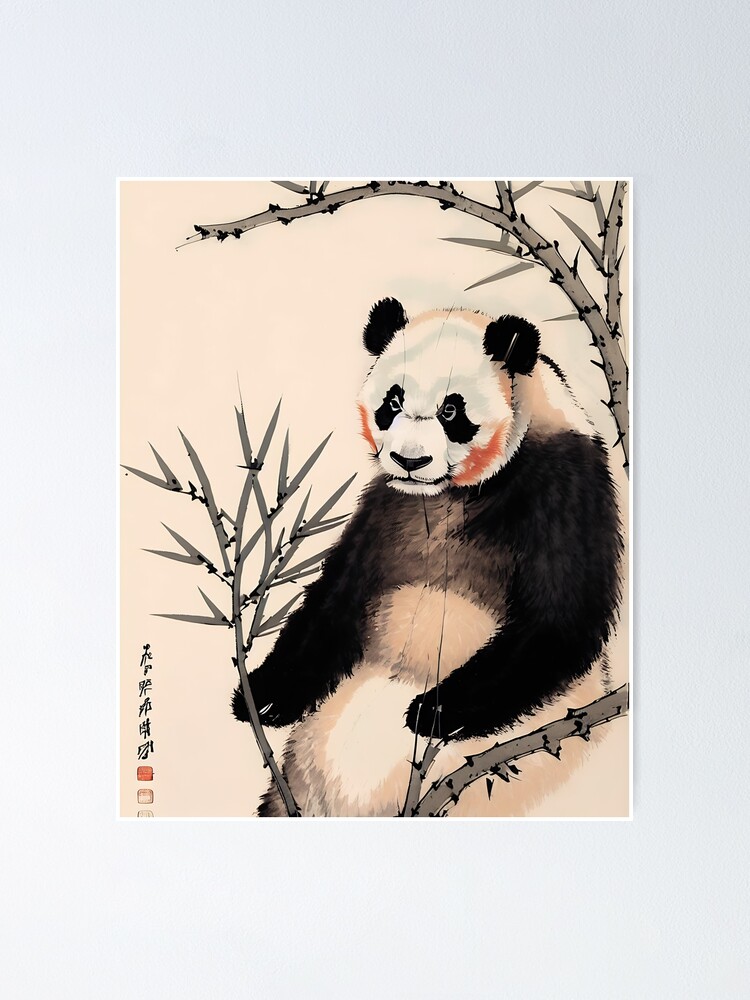This rectangular illustration features a detailed depiction of a classic black and white panda bear with small, rounded black ears and distinctive black fur around its eyes. The panda, rendered with red-tinged cheeks adding a soft touch of color, is positioned on the right side of the image, gazing towards the center left. Its long arms, complete with claws, rest on its stomach. The panda is surrounded by bamboo branches and leaves, with one branch arching over its head and others around it. The background of the illustration is a very light, reddish-white color, contrasted by the gray matte framing the entire image. In the lower left corner, there are Asian characters, likely the artist's signature, adding an authentic touch to the scene. The overall effect is reminiscent of a stamp, blending traditional art styles with a warm, charming depiction of the panda in its natural habitat.